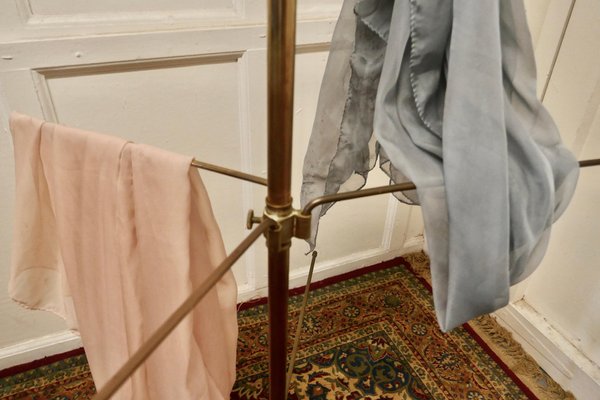In a corner of an indoor room, there's a tall pole stretching up from a heavily dirtied rug that features ornate, floral patterns in red, green, beige, and light beige hues. The rug, which has fringes at the ends, closely resembles a Persian or Turkish design. At the base of a white wall, where it meets the floor, dirt accumulates prominently at the trim. 

The central structure in the scene is a bronze or brass clothes drying rack. This rack consists of a main vertical pole with several arms extending outwards. On the left arm, a sheer, peach-colored fabric hangs delicately. Higher up, on the right side, a similarly sheer fabric in a light gray color is draped. There's also a thin blue piece of clothing, possibly a shirt or dress, hanging on the right side of the rack. The white wall behind features some wooden decoration and appears grimy, especially in the corners and around the trim, adding to the room’s unkempt appearance.